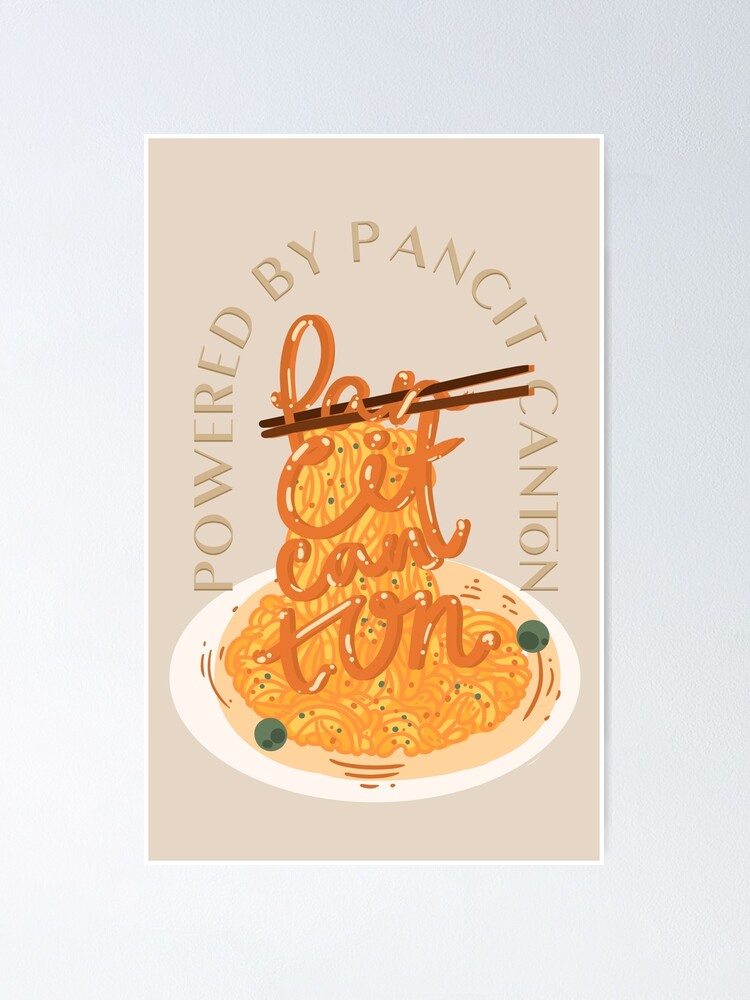The image is a vertical, portrait-oriented vector illustration set against an almost grayish background with a very narrow white border. Inside the border, the main illustration features a cream-colored plate filled with vivid yellow and orange noodles, representing the Filipino dish, Pancit Canton. The plate is adorned with two small, dark olives or calamansi on either side. Scattered across the noodles are tiny green and red flecks, possibly pepper flakes or basil, adding a touch of color and hinting at the dish's flavor. 

Across the top of the plate, in an arched style resembling a doorway, is the text "Powered by Pancit Canton" in brownish-tan lettering. In the center of the illustration, bright red text spelling "Pan" appears to be held aloft by a pair of red chopsticks, with "Pancit Canton" written beautifully beneath it in a cursive-like font that mimics the noodles' texture. This integrated presentation not only highlights the dish but also conveys a traditional and cultural essence, achieved through both typography and illustration.